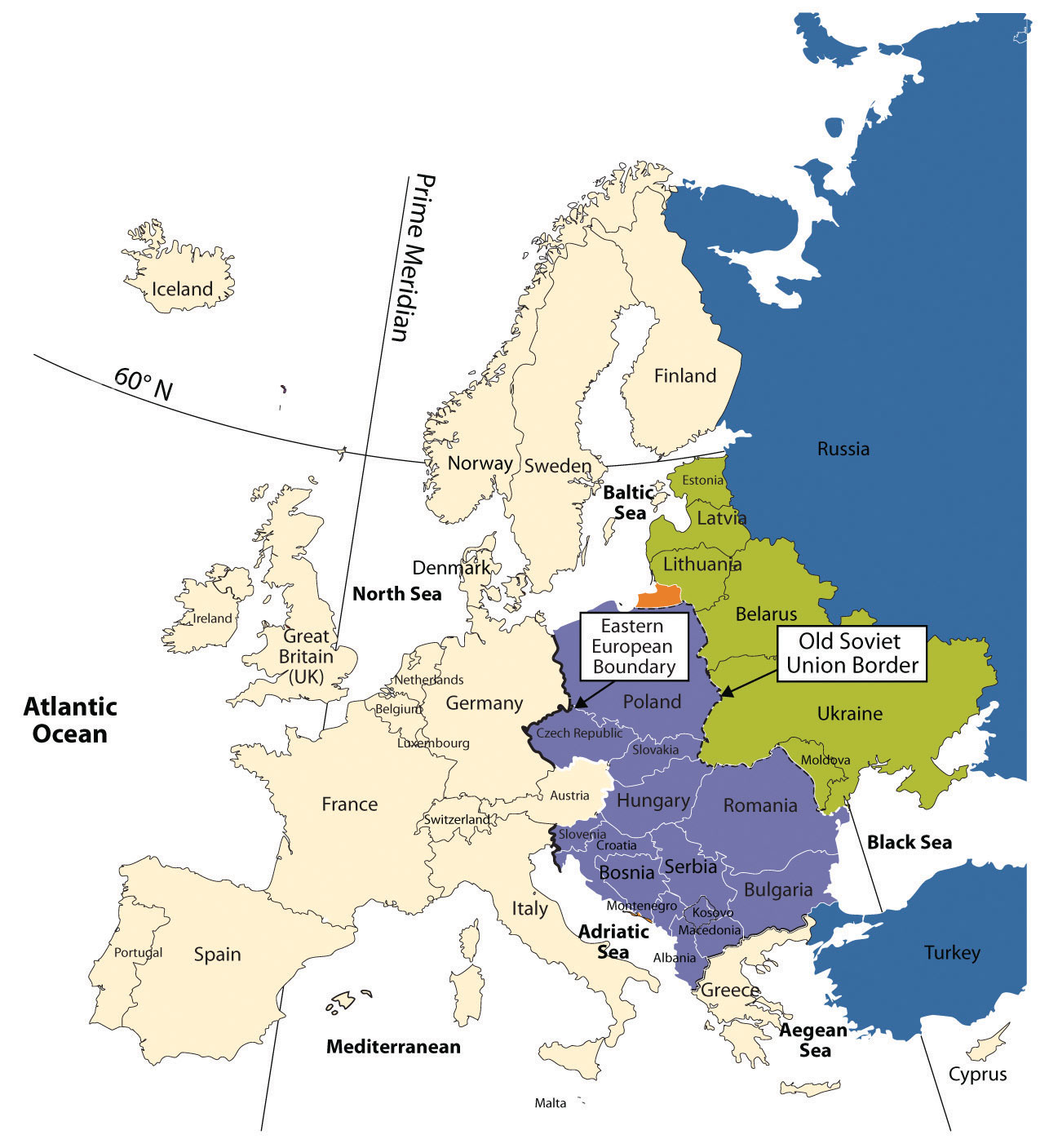The image is a detailed map showcasing various parts of Europe and its surrounding areas. On the far left is the Atlantic Ocean, depicted against an all-white background. The map prominently features a curved line labeled "60 degrees north" descending from the upper left towards the center. Diagonally from top to bottom, a slanted line labeled "Prime Meridian" is also visible. In the upper left corner, the outline of Iceland is highlighted in pink. Below that, Spain and Portugal are similarly outlined in pink. Moving rightward, adjacent to the Prime Meridian, the map labels the Mediterranean Sea in black.

A cluster of countries, also colored in pink, spans upwards from Spain through France, Germany, and up to Norway, Sweden, and Finland. The right side of the image is dominated by Russia, emblazoned in black on a large blue area. Underneath Russia, several countries, including Estonia, Latvia, Lithuania, Belarus, and Ukraine, are depicted in green. The old Soviet Union border is indicated by a rectangular cutout with an arrow pointing to the edge of Ukraine and Poland.

Beneath the green section is a purple-hued region containing Poland, Hungary, Romania, Bosnia, Serbia, and Bulgaria. In the lower right-hand corner, Turkey appears in blue with "Turkey" labeled in black, just above Cyprus, which is marked by a small pink patch. Additional details include the Black Sea below Ukraine and Turkey, the Aegean Sea to the left of Turkey, and Greece above the Aegean Sea. Further left, the Adriatic Sea is shown beside Italy's characteristic boot shape.

The map intricately combines multiple geographic details, providing clear distinctions between countries and seas, showcasing the diverse regions of Europe and parts of the surrounding areas.